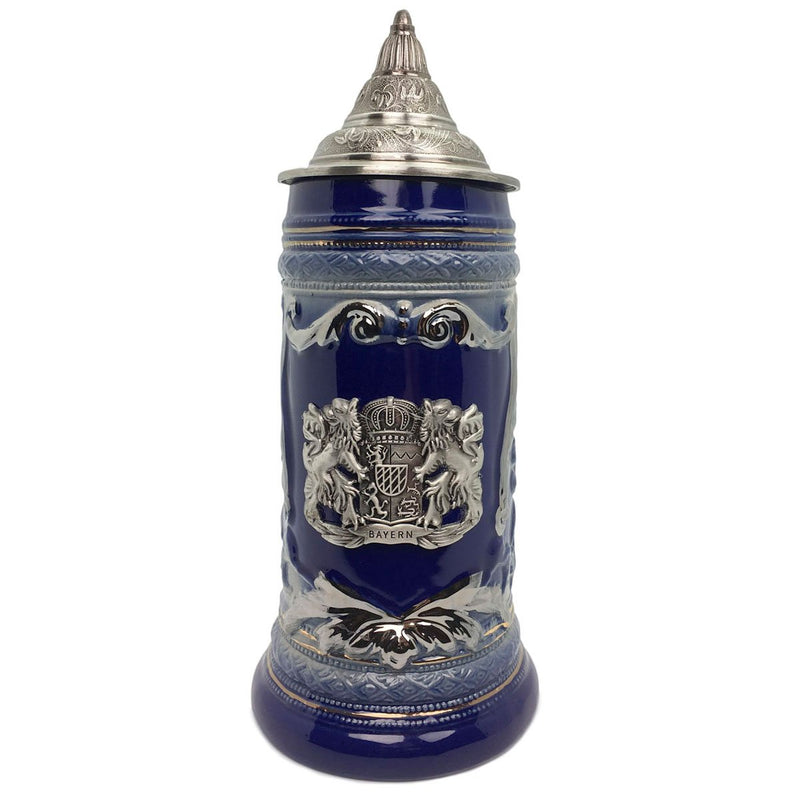The image depicts a close-up view of a highly detailed and ornate container, possibly an urn, vase, or beer stein. This elegant piece features a navy blue body adorned with intricate silver designs. The navy blue surface is embellished with a prominent silver emblem that evokes a medieval aesthetic, resembling a family crest. The crest includes two lions facing each other, flanking a central shield topped with a crown, and inscribed with the word "Bayern." The emblem is surrounded by an ornate border that resembles embroidery, contributing to its elaborate appearance.

The design extends into patterns of cross-hatching and 3D floral or leaf motifs that complement the central emblem. The bottom of the container is encircled with silver, possibly reflecting light to give the appearance of gold rings. The container is topped with a silver dome that has an engraved, triangular design, reminiscent of a capitol building dome. While the material appears ceramic at first glance, the thickness and reflective quality suggest it might be crafted from a solid, heavy metal. The background of the image is either white or non-existent, focusing attention entirely on the intricate details of the container, which is closed, revealing nothing of its interior.